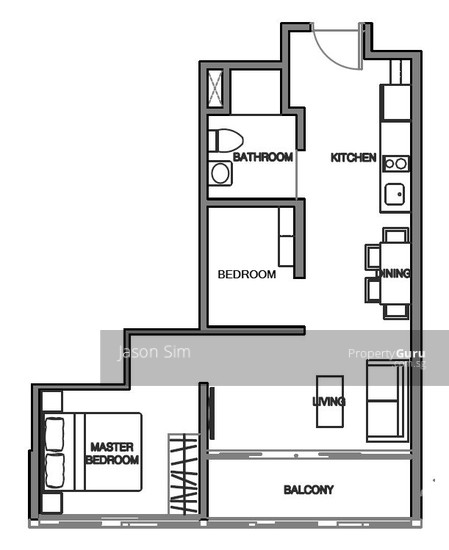Detailed Caption:

This blueprint showcases a detailed floor plan, likely of a single-level residence given the absence of indicators for multiple levels. Centrally featured is a spacious balcony adjacent to the master bedroom, which includes a designated closet area. Exiting the bedroom leads directly into an open living space.

From the balcony area—partially connected to the living space—the blueprint prominently displays the name "Property Guru" and "Jason Sim," suggesting it might be the property listing or brokerage details. Transitioning from the living space, one enters the dining room, which is positioned adjacent to an additional bedroom.

Beyond the dining area, the layout flows into the kitchen, clearly marked with defined counter areas, including the sink. Neighboring the kitchen is a large powder room, equipped with a sink and toilet but notably lacking a shower. Past this powder room is an open space leading back to a door that provides another entrance into the kitchen.

Throughout the blueprint, the exterior walls are delineated in a bold gray line, while the interior lines are rendered in a lighter gray, highlighting the meticulous planning of the space's segmentation. Additionally, there is a peculiar feature marked by two lines that may represent a closet or a similar storage area, although its exact purpose remains ambiguous.